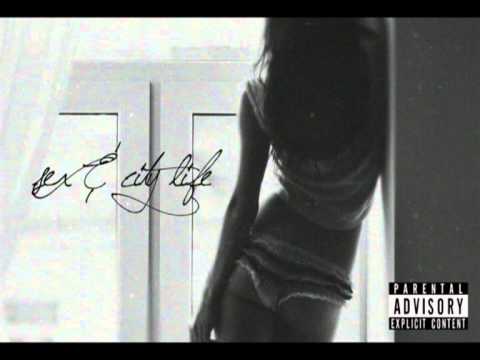The image is a black-and-white cover, likely for an album or a DVD, titled "Sex & City Life," written in cursive letters on the left side. A Parental Advisory Explicit Content label is positioned in the lower right corner. The main focus is a scantily clad woman with long hair, wearing a very light shirt and short panties, showcasing her back and buttocks. She leans against a wall and gazes out of a window with curtains, looking toward the horizon. The window appears to lead to either double doors or another doorway. The combination of the handwritten title and the subtle, provocative imagery contributes to a sophisticated yet edgy aesthetic.